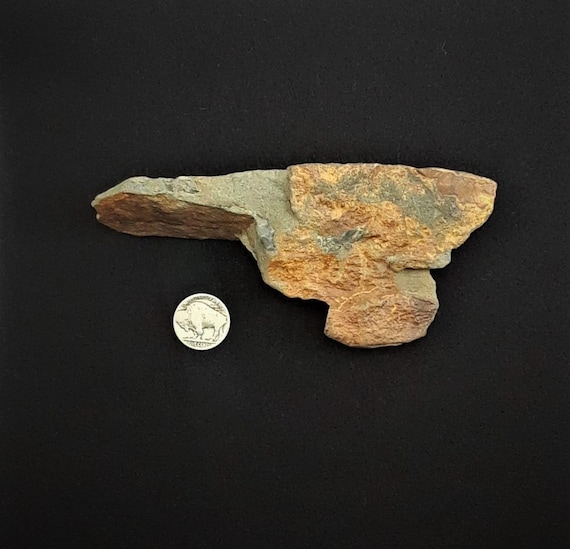The image features two objects: a rock and a coin, set against a plain black background that accentuates their colors and textures. The rock, which is the larger of the two objects, is uniquely shaped like a gun, with its long end pointing to the left. It has a varied coloration, transitioning from bronzish orange to gray, creating the appearance of a weathered cliff face. The coin, a silver buffalo nickel, is positioned down and to the left of the rock. The vivid contrast between the metallic shine of the nickel and the earthy tones of the rock highlights the distinct textures of both items. The background simplicity and the relative position of the objects enhance the rock’s unique shape and the coin’s intricate detailing, with the buffalo and inscriptions faintly visible.